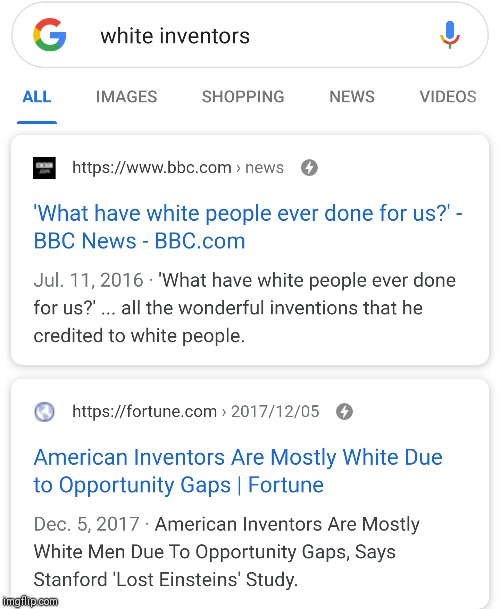Here is the polished and detailed description:

This screenshot captures a portion of a Google web search. The background of the screenshot is entirely white. In the lower left-hand corner, there is a watermark indicating that this image is hosted on "imgflip.com." 

In the upper part of the screenshot, the Google search bar is prominently displayed. To the left of the search bar, there is a colorful 'G' logo, characterized by its red, yellow, green, and blue shades. Inside the search bar, the phrase "white inventors" has been typed. On the right side of the search bar, there is a microphone icon, signifying the option to conduct a voice search.

Below the search bar, the "All" search tab is selected, evidenced by the tab being highlighted in blue text with a blue line underneath it. 

The first search result listed is from BBC.com, with the headline, "What Have White People Ever Done for Us?" dated July 11, 2016. The description accompanying the headline states, "What Have White People Ever Done for Us? All the wonderful inventions that he credited to white people."

The second search result is from fortune.com, with the title, “American inventors are mostly white due to opportunity gaps,” dated December 5, 2017. The description mentions, "American inventors are mostly white men due to opportunity gaps, says Stanford. Lost Einstein Study."

Overall, the screenshot provides a visual snapshot of a Google search query related to the topic of white inventors, along with associated search results.